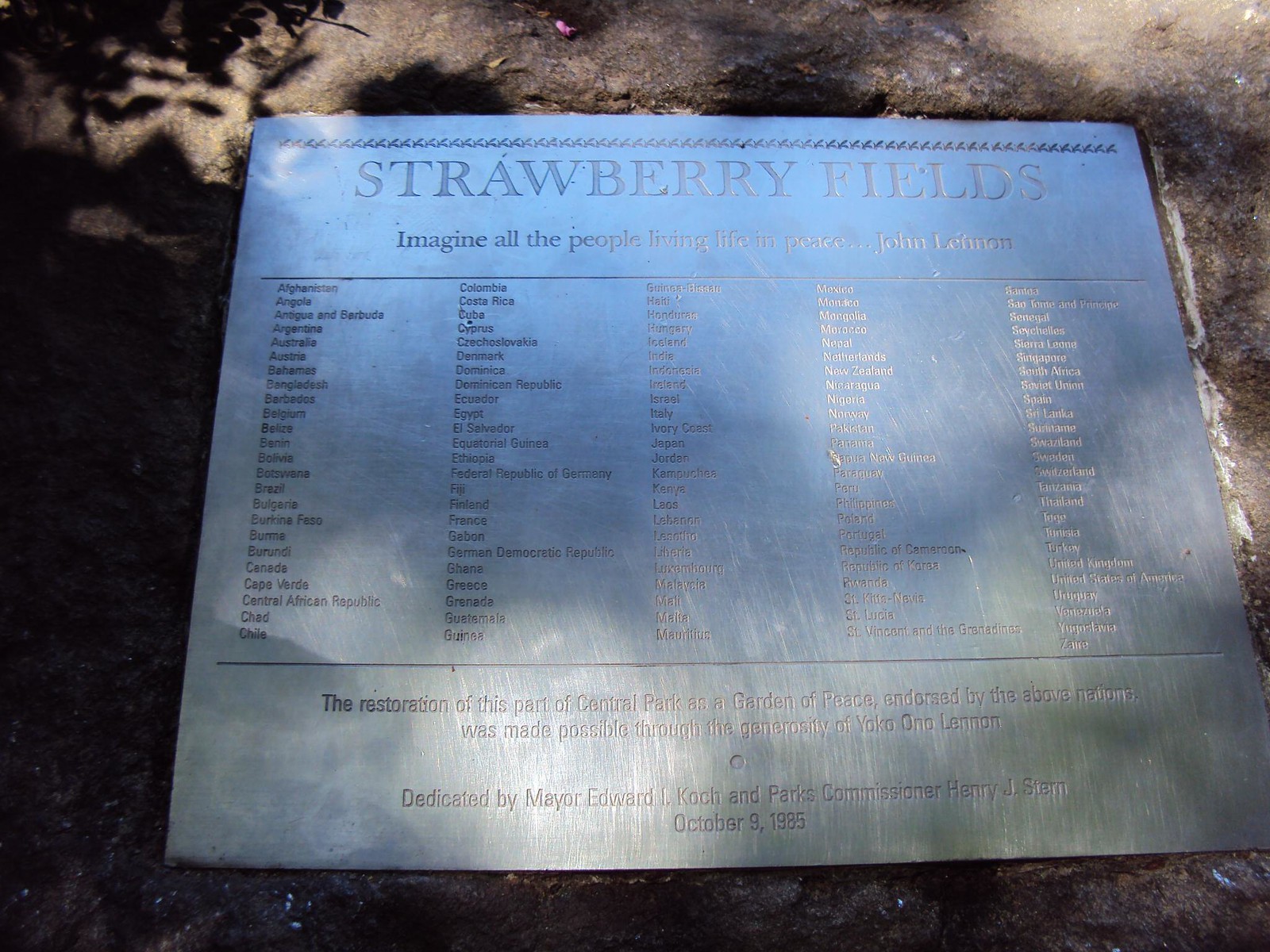This image captures a beautifully crafted plaque set in Central Park, New York, surrounded by a grassy backdrop. The plaque is dedicated to "Strawberry Fields," in tribute to John Lennon, and bears the line from his iconic song, **“Imagine All the People Living in Perfect Peace.”** This dedication—a vision of global harmony—is reinforced by a list of participating countries arrayed in columns. The first column begins with Afghanistan and Chile, while the subsequent columns list Colombia, Cuba, Denmark, and others, reflecting a diverse international endorsement of peace. Beneath this, the plaque mentions its restoration as a garden of peace, made possible through the generosity of Yoko Ono Lennon, highlighting her commitment to her late husband’s legacy. The dedication, commemorated by Mayor Edward Koch and Parks Commissioner Henry J. Stern, is dated October 9, 1985. The plaque, though scuffed and weathered by time, shines under bright sunlight, making some details difficult to discern. Despite this, its message of peace endures, harmonizing beautifully with its natural setting.